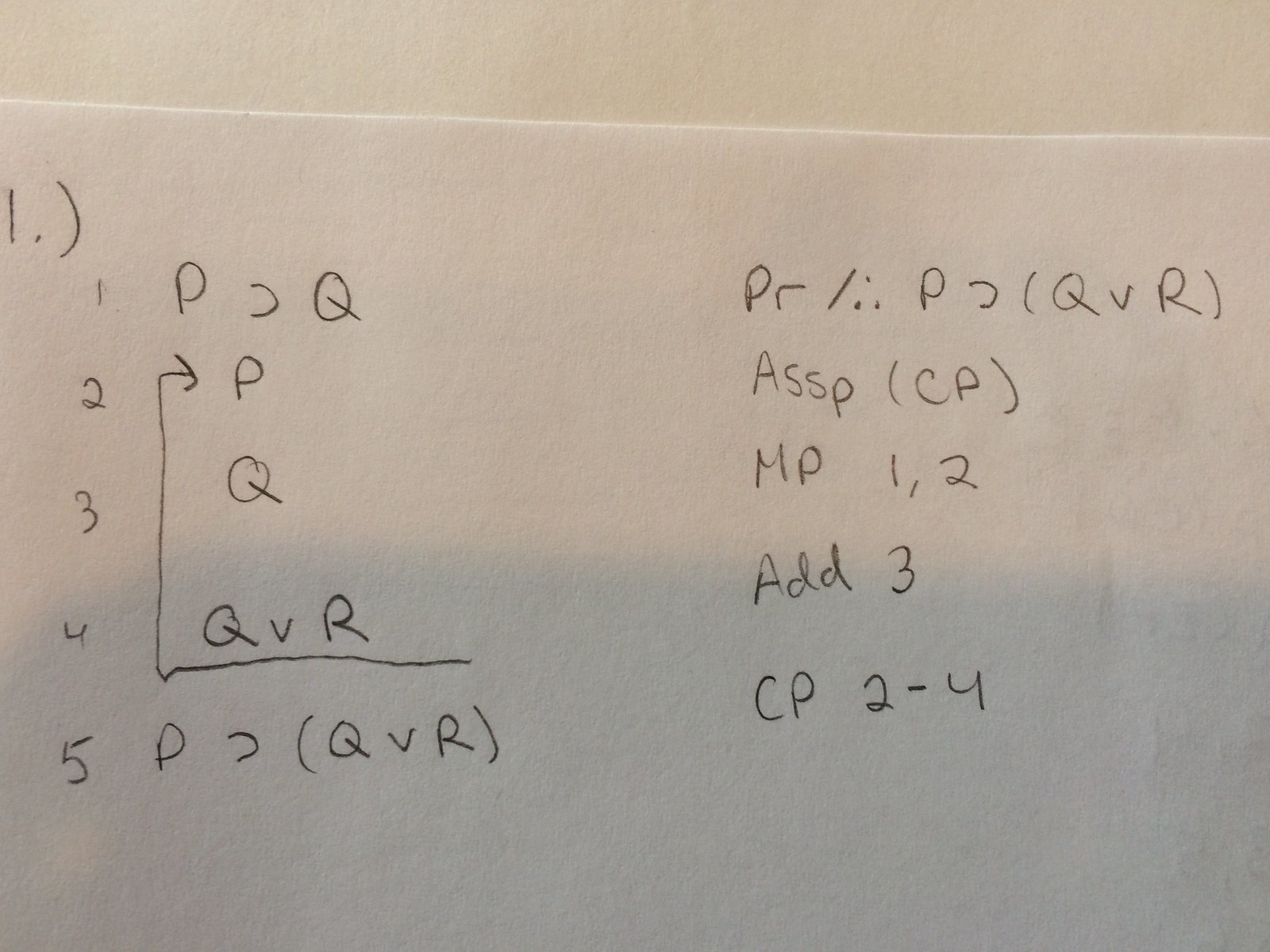This photograph captures a sheet of white or slightly off-white paper, positioned on top of another paper. Featured on the paper is a written math problem, labeled as "Problem Number 1." The problem is structured into five cryptically denoted steps, arranged in two parallel columns. 

In the first column:
1. \( P \mathrel{\backepsilon} Q \)
2. \( p \)
3. \( Q \)
4. \( Q \lor R \)
5. \( P \mathrel{\backepsilon} (Q \lor R) \)

The corresponding steps in the adjacent column are more complex:
1. \( PR \slash \therefore P \mathrel{\backepsilon} \forall Q \lor R \forall N \)
2. \( ASSP(CP) \)
3. \( M P_{1,2} \)
4. \( \text{Add 3} \)
5. \( CP_{2-4} \)

The mathematical symbols and notations suggest an advanced or abstract mathematical proof or solution. The layout indicates that each step in the first column has an associated, albeit cryptic, explanation or extension in the second column.